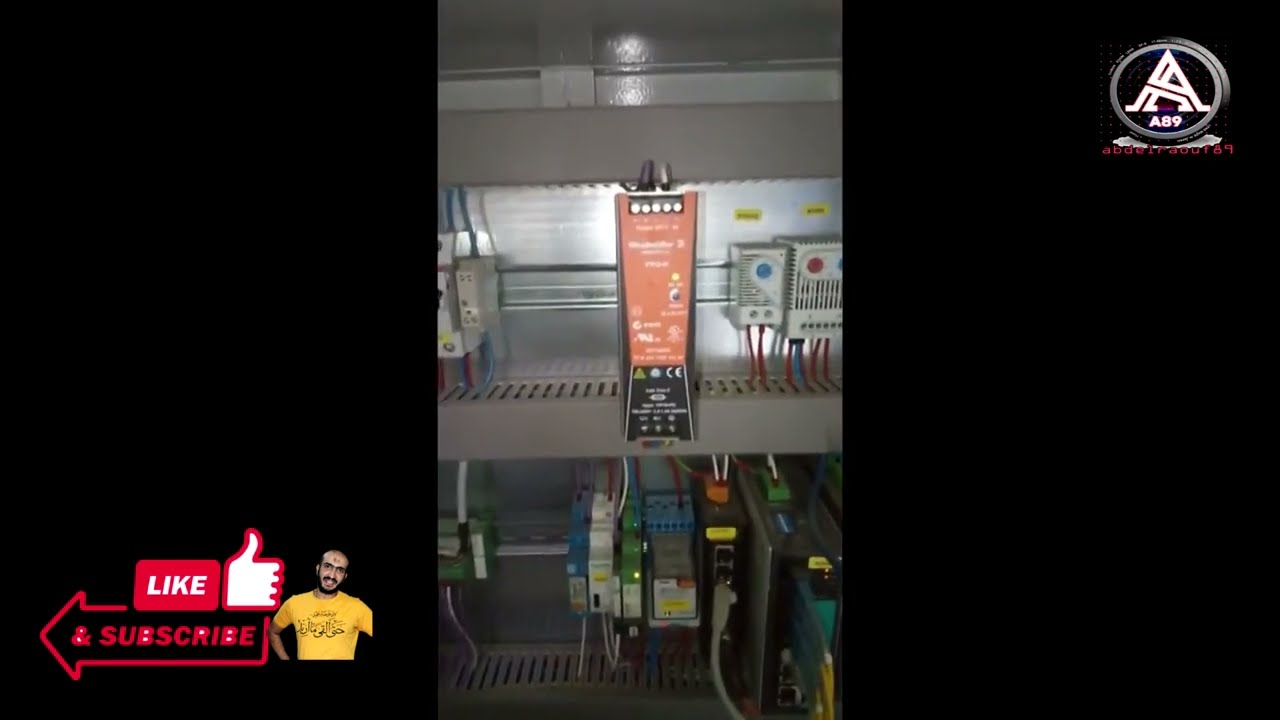The image appears to be a composite photograph from a social media channel, divided into three sections. The left third of the image features a black background with a red "Like" button, depicted as a thumbs-up icon within a red rectangle. Beneath this, in another red arrow shape, is the prompt to "Subscribe." Nearby stands a man, likely of Indian descent, dressed in a yellow shirt, smiling at the camera. The center section of the image showcases an electrical or network junction box. This compartmentalized space is filled with a variety of electronic devices, possibly routers or network switches, indicated by multiple Ethernet cables plugged in and various colorful components like blue, green, red, and white. The shelves within the box have slats or grid lines, allowing for organized cable management. The right third of the image again displays a black background, featuring an upper right logo—a gray circle with a white, double-stacked 'A' labeled as "A89"—positioned within a black square adorned with yellow grid-pattern dots and red alphanumeric code "A B D C E F 2001 8 9".